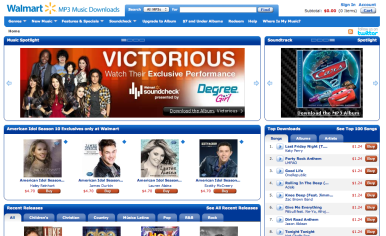The webpage of Walmart prominently features the Walmart logo in blue letters at the top with a blue and white color scheme. Beside the iconic yellow Walmart logo, it reads "MP3 Music Downloads." There is a search bar specifically for MP3s, along with options to sign in, access your account, and view your cart for potential purchases. 

Dominating the page is a large promotional image of the band Victorious. The word "VICTORIOUS" is displayed in bold white, capitalized letters. Beneath this, in smaller white text, it invites users to "watch their exclusive performance," highlighting a Soundcheck performance. There is also an option to download their song. Additionally, the text "Degree Girl" appears, with "Degree" in blue letters and "Girl" in pink.

Adjacent to this, there's a feature on the Cars soundtrack, showcasing a picture of characters from the movie Cars alongside the recognizable Cars logo set against a thematic background. Further down, there are options to purchase MP3s from various American Idol seasons. The webpage categorizes other music releases into genres like Children, Everyday, Pop, R&B, among others, available for purchase.

On the right-hand side, there's a section titled 'Top Downloads' listing the most popular songs and albums. It lists eight top downloads along with their durations and provides the option to buy these MP3 songs.